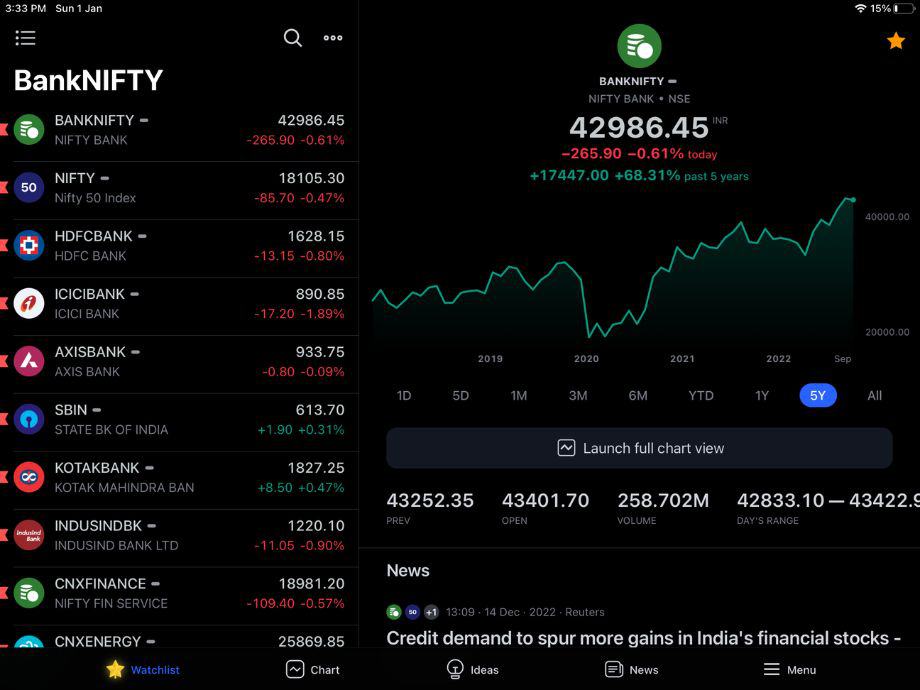This image is a screenshot captured from a mobile phone displaying an investing app named "Bank Nifty." At the top of the screen, the status bar shows the current time, date, full Wi-Fi signal, and a 15% battery charge. The app is focused on banking and financial stocks.

On the left-hand side, there is a vertical list of various banks and financial institutions, each accompanied by their respective logos in circular icons. The listed entities include: Bank Nifty, Nifty, HDFC Bank, ICICI Bank, Axis Bank, SBIN, KOTAK Bank, IndusInd Bank, CNX Finance, and CNX Energy.

To the right of each bank or financial institution name, trading information is displayed, showing current prices and whether they have gone up or down. In the central section and extending towards the right, a prominent display reads "Bank Nifty" and "Nifty Bank NSE," with a current value of $42,986.45, indicating a decline of $265.90.

Below these figures, there is a line graph showing the performance of the investments over a five-year period, as indicated by the "5Y" marker being highlighted. At the bottom of the screen, a headline reads, "Credit demand to spur more gains in India's financial stocks," suggesting positive future performance in the sector.